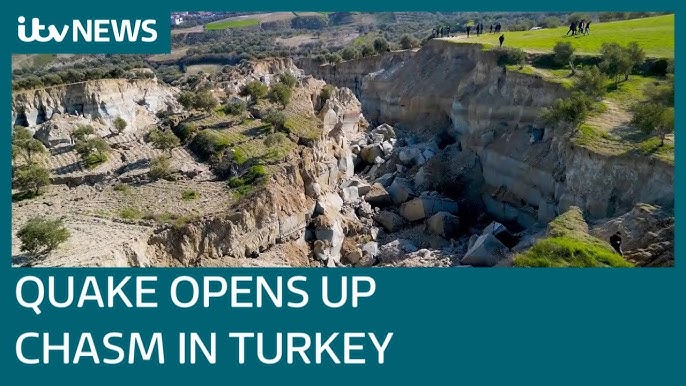The image features a news graphic with a blue background. At the top left, white text reads "ITV News," and at the bottom, another white text states "Quake opens up chasm in Turkey." The picture shows a deeply split earth, indicating a massive chasm formed by an earthquake. On the right side of the chasm, the terrain is covered in smooth, lush grass that resembles a well-kept field. The left side contrasts with a rough, dirt-laden area scattered with boulders and rocks that have crumbled into the chasm. Large sections of the earth appear to have split and fallen, with people standing at the edge and others walking around, inspecting the massive rift. The chasm stretches deep into the valley floor, highlighting the significant impact of the earthquake.